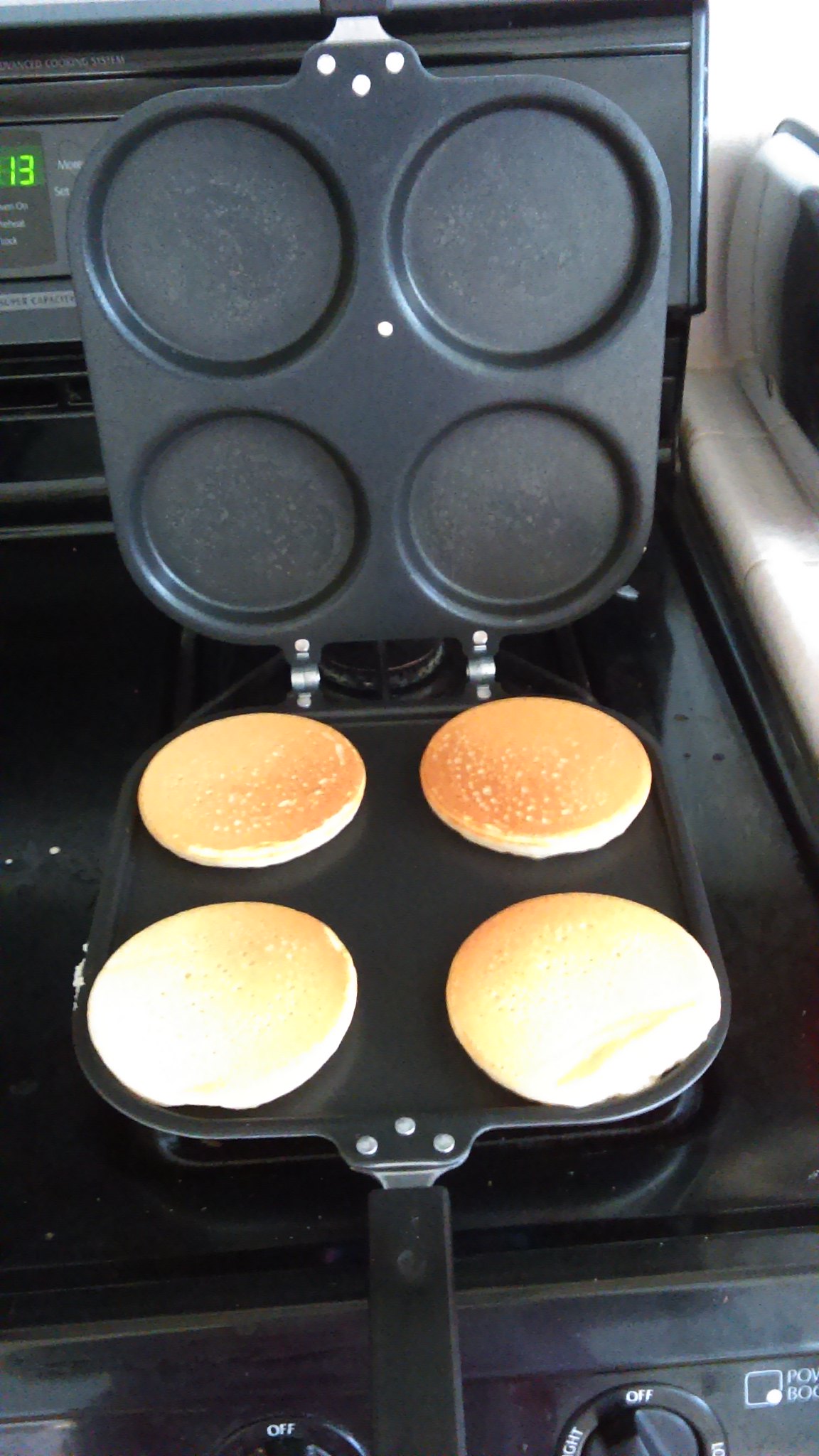In this detailed photograph of a kitchen, a four-slot pancake maker sits prominently atop a stove. The black pancake maker, which has a griddle with four circular molds for perfectly shaped pancakes, is currently open, revealing its freshly cooked contents. The two pancakes at the top are a golden brown, indicating they were cooked slightly longer than the two at the bottom, which are a lighter shade. The sturdy black pan has a flat bottom and a top section with cut-out circles to shape the pancakes, complete with hatches that allow flipping. The stovetop beneath the pancake maker shows partial views of two knobs, one of which appears to be turned on. In the background to the right, on the white tile countertop, an indistinct device can be seen, though it is unclear whether it is a toaster or something else, as the image cuts off too quickly to identify it precisely.